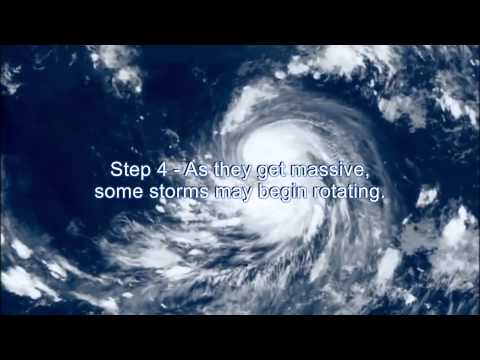This overhead image captures the swirling formation of a hurricane, centered prominently amidst a vast expanse of blue, likely representing the ocean. The hurricane is characterized by a distinctive white cloud formation with a noticeable tail extending towards the left corner, and is flanked by additional clouds in both the upper and bottom right corners. Across the middle of the image, white text reads, “Step 4. As they get massive, some storms may begin rotating,” lending to its educational vibe, potentially as a screenshot from a radar tracking system or a weather channel broadcast. The image also features black strips at the top and bottom, suggesting it might be viewed on a mobile device or tablet. The overall aesthetic points towards an instructional setting, possibly used to teach about storm behaviors like hurricanes or tornadoes.